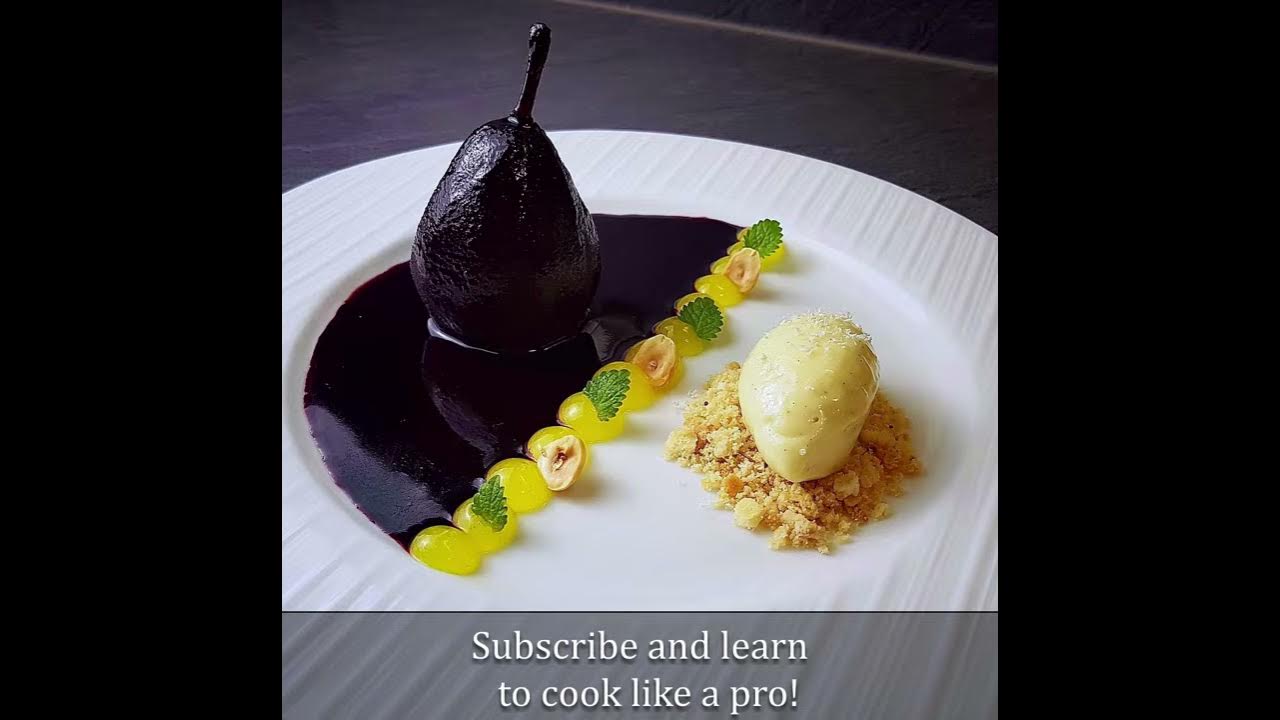This detailed and descriptive caption showcases the combined details from each voice input:

In this enticing image, we see a sophisticated culinary dish artfully plated on a white circular plate with a textured rim. The plate rests on a dark surface, framed by two black bars suggesting it might be a still from a video. The dish itself presents a striking contrast with bold colors and intriguing textures, inviting a double-take.

On the left side of the plate, there's a pear-like fruit, entirely cloaked in a deep, tar-like purple or black substance, with a stem poking gracefully upwards. This part of the dish sits in a small puddle of the same purple liquid. The visual impact is enhanced by the dramatic coloring and aesthetics, as if the pear has been dipped in a mysterious culinary concoction.

Separating this dark, enigmatic presentation from the right side is a neat line of small, yellow, marble-like candies or grapes, each adorned with delicate decorations such as tiny leaves or halves of peanuts. These vibrant yellow elements add a burst of color to the composition and serve as a transition to the more subdued right side of the dish.

To the right, a sophisticated dessert awaits. A mound of finely crunched breadcrumbs forms the base, atop which sits a dollop of creamy, beige substance. It might be ice cream or some other delicate cream dessert. Clear flakes, possibly sugar or salt, are sprinkled on top, suggesting a delightful texture contrast in every bite.

The background of the image is minimalistic—only a glimpse of the dark surface beneath the plate can be seen, directing all focus to the culinary masterpiece. At the bottom of the image, a caption invites viewers to "Subscribe and learn to cook like a pro," hinting that such exquisite creations can be within reach.

With carefully balanced elements and a composition that plays with color and textures, this dish is more than a meal; it's a piece of art waiting to be savored.